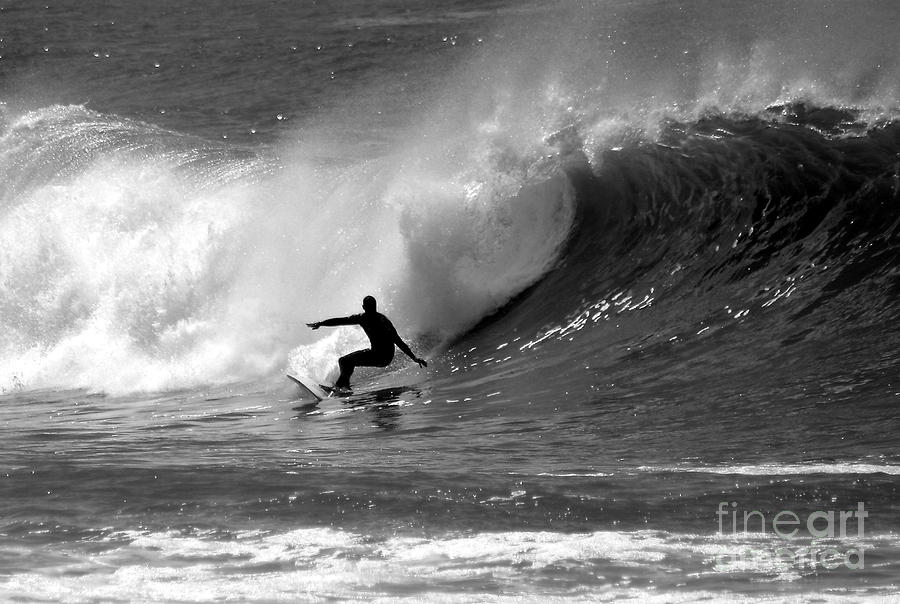A captivating black-and-white high-resolution photograph captures a surfer silhouetted against a massive, tunnel-like wave. The surfer, likely male, is in a crouched position with arms outstretched and legs bent, expertly balancing atop a surfboard. He is positioned right in the midst of the rolling wave, with ocean spray cascading from its crest. In the foreground, breakers add to the dynamic energy of the scene. A watermark in the bottom right corner reads "Fine Art," though the rest is obscured as it blends into the white waves. This striking image evokes classic California or Hawaii surfing moments, enhanced by glistening highlights in the water.